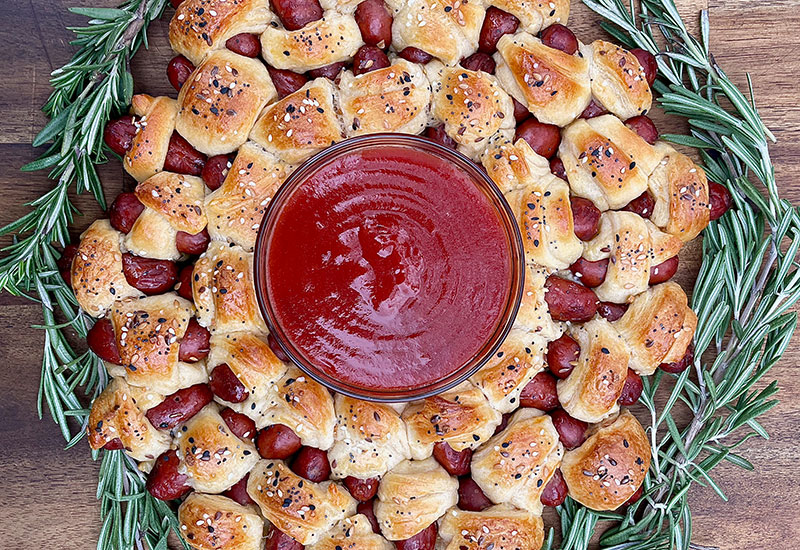This is a detailed bird's-eye-view photograph of a festive platter featuring layers of appetizers known as pigs in a blanket. Arranged in a circular fashion on what appears to be a wooden table, these savory treats are baked to a golden brown and sprinkled with sesame seeds. Each pig in a blanket consists of a small hot dog wrapped in bread dough. In the very center of this mouthwatering display is a clear bowl filled with a vibrant red dipping sauce, likely ketchup, designed to complement the appetizers. A wreath of twigs, peppered with decorative herbs such as rosemary, encircles the outer layer, adding an elegant touch to the presentation. Additionally, part of a different plant can be seen on the fringes of the food setup, enhancing the aesthetic appeal. The image, captured from a high angle, vividly showcases the intricate details and textures of both the food and the surrounding elements, making it look deliciously inviting and perfect for any party.